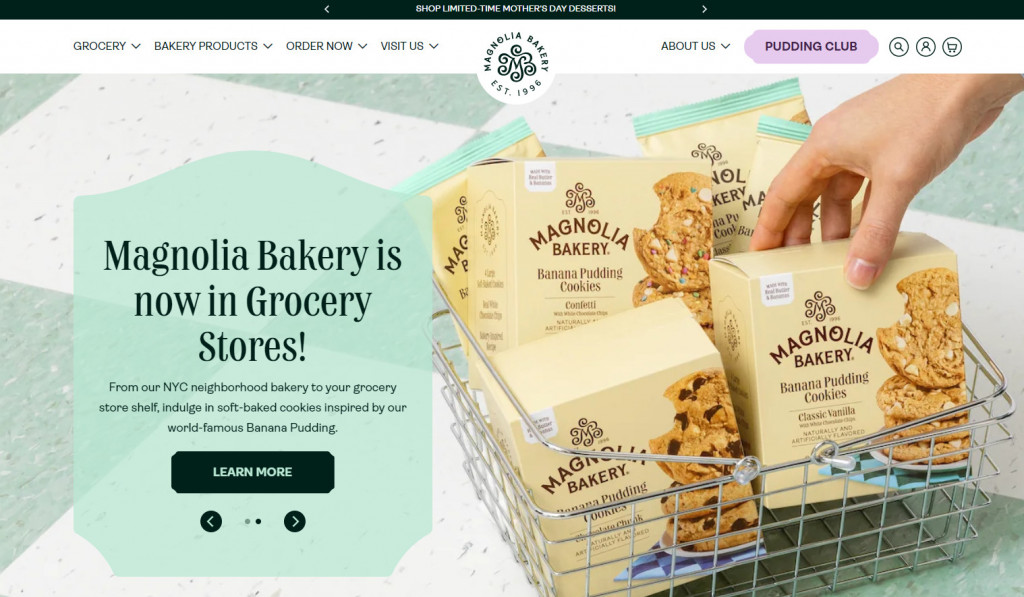The web page features a dark navigation bar at the top, showcasing options such as back and forward arrows, and a central message proclaiming "Shop limited time Mother's Day desserts". Below this is a white and light green bar with drop-down menus labeled "Grocery," "Bakery Products," "Order Now," and "Visit Us." 

A detailed logo for Magnolia Bakery, established in 1986, is prominently displayed. To its right are links for "About Us," a "Pudding Club" purple button, a search icon, and icons for account management and shopping basket.

The main image features a green and white checkered tablecloth with a gray banner announcing, "Magnolia Bakery is now in grocery stores." It highlights the journey from their New York City bakery to grocery store shelves, offering indulgent soft-baked cookies inspired by their world-famous banana pudding. An inviting "Learn More" button is available for additional information. The image showcases a variety of cookies, including one being placed into a basket, emphasizing the delicious appeal of banana pudding cookies, reminiscent of Southern flavors.